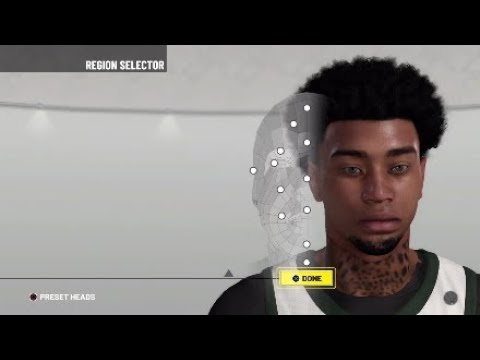A screenshot captures a video game loading screen, likely for a basketball game, prominently featuring a region selector menu. The focal point is an African-American male character with a modest Afro and a neatly trimmed goatee. He is dressed in a white basketball jersey layered over a black shirt, showcasing tattoos on his neck. The background of the screen is mostly obscured but includes a black bar at the top and bottom of the image, likely indicating a widescreen format. There is a yellow "close" menu displayed, though the text is illegible. The overall scene appears to be photographed from a TV, creating a slightly reflective white wall backdrop in the room behind.